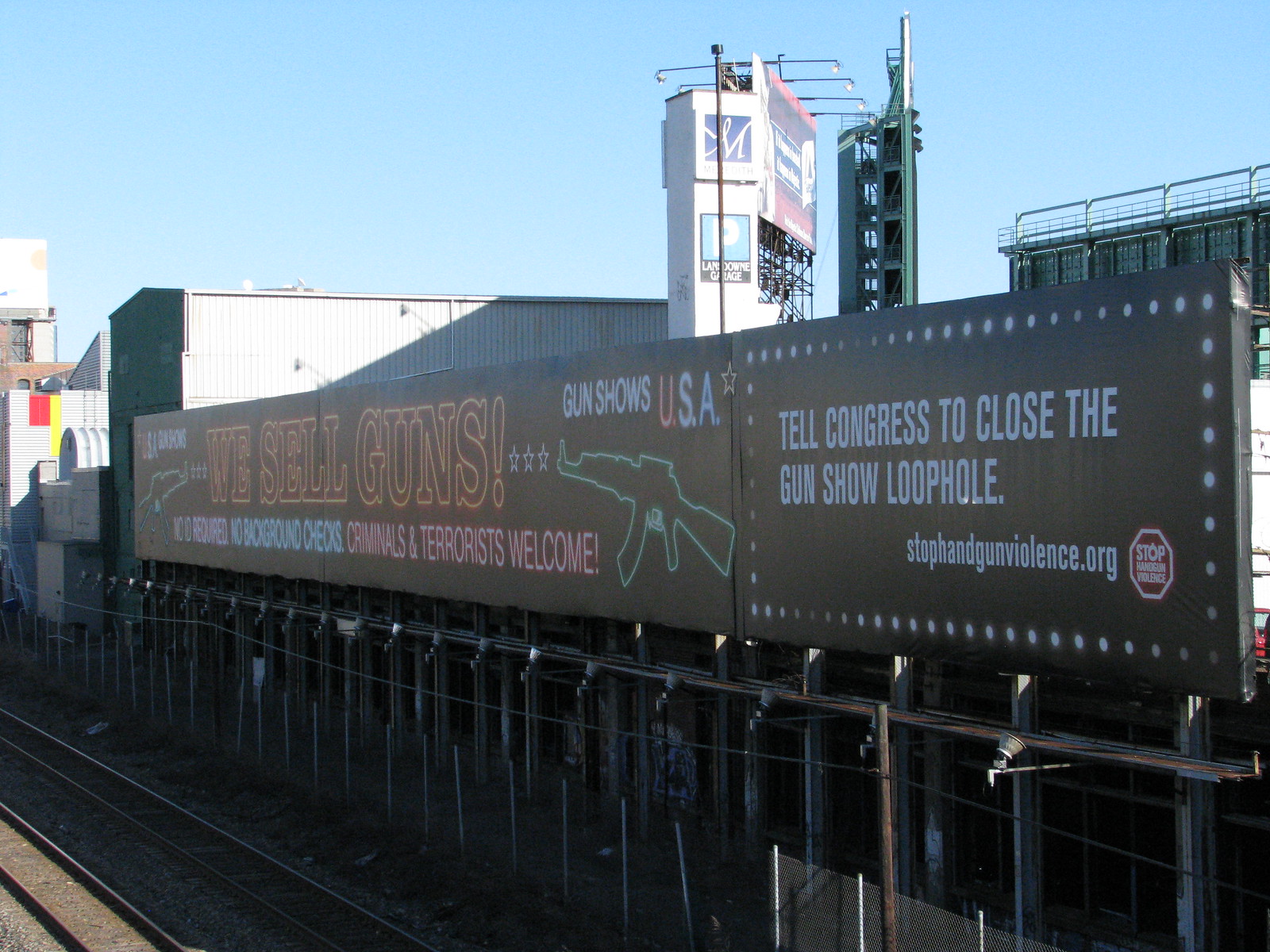In the outdoor image, large billboards dominate the scene. In the bottom left corner, train tracks are visible, partially obscured by a chain-link fence that lines the area. Supporting the billboards are sturdy posts. To the left of the billboards stands a white-colored building, extending halfway through the image and rising above the billboard's height. A clear, blue sky forms the backdrop.

The primary billboard is long and rectangular with a black background, divided into two sections: the right section and the left section. The right section, taking up about a third of the total space, features white text urging, "Tell Congress to close the gun show loophole. Stophandgunviolence.org." This message is complemented by a red stop sign with a border of circles, enhancing its call to action.

The left section of the billboard, larger and more prominent, contains bold letters declaring, "We sell guns. Gun shows USA." Illustrated in green are several guns. Below, though partially obscured and hard to read, the text seems to provocatively state, "No background checks, criminals and terrorists welcome." The juxtaposition of these messages starkly highlights the conflict between advocacy for gun control and the promotion of gun sales without restrictions.